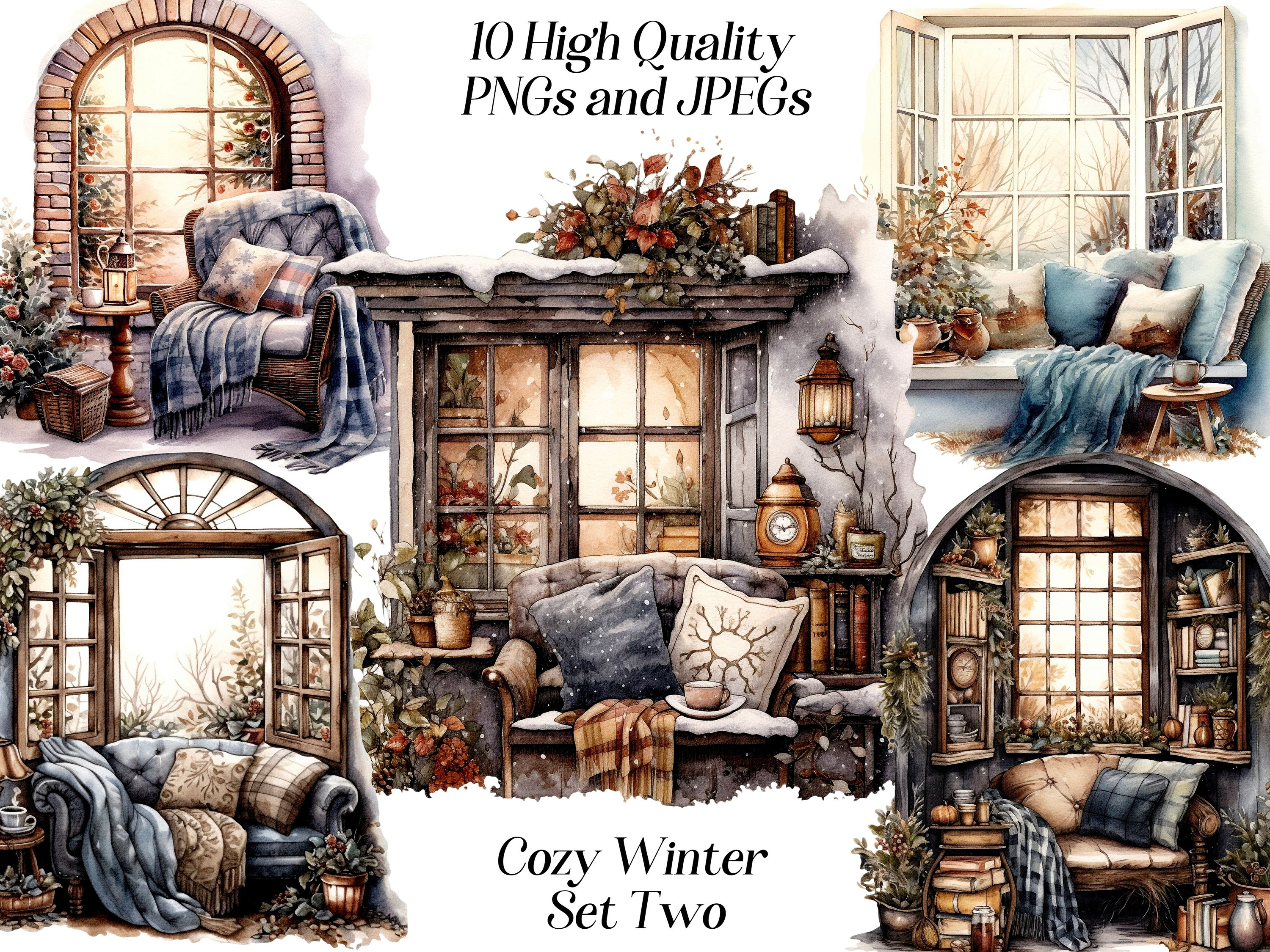The image features a cozy winter-themed set of five high-quality PNG and JPEG illustrations, with black text at the top stating "10 high-quality PNGs and JPEGs" and "Cozy Winter Set 2" at the bottom. Each illustration showcases a different window scene, each with unique seating arrangements facing outwards. One corner depicts a window with a chair adorned with a blanket, pillows, and a small side table. Another shows a window seat, similarly outfitted with a blanket, pillows, and a table in front. The center illustration highlights an armchair with pillows, a blanket, and a cup and saucer in front of the window. A bottom corner features a wooden chair with pillows beside shelves. The final corner has a love seat with pillows, two blankets, and an open window looking outside. All scenes are decorated with night lamps, teapots, books, coffee mugs, and an abundance of flowers and plants, contributing to an overall cozy, wintry atmosphere.